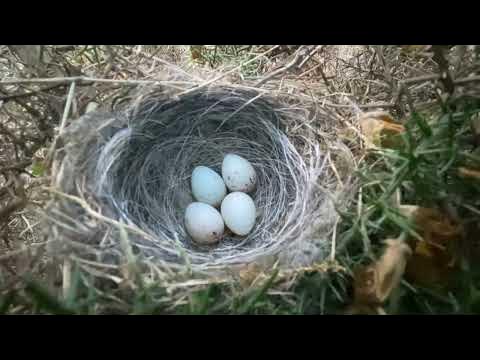This landscape-oriented photograph features a carefully framed image of a bird's nest, bordered by horizontal black bars at the top and bottom. The nest, nestled within a bush or thicket rather than high in a tree, is a beautifully constructed round bowl made from a mixture of twigs, grasses, straw, and a few little feathers. It is intricately woven, displaying an artistic combination of whitish, tan, and brown materials, with some grayish-white weavings in the center. The scene is decorated with green and brownish leaves. Looking down into the nest, we see four speckled eggs, light in color, varying from bluish-white to gray, some with black smudges. There are no birds in sight, which brings all the attention to the detailed craftsmanship of the nest and the delicate eggs within.